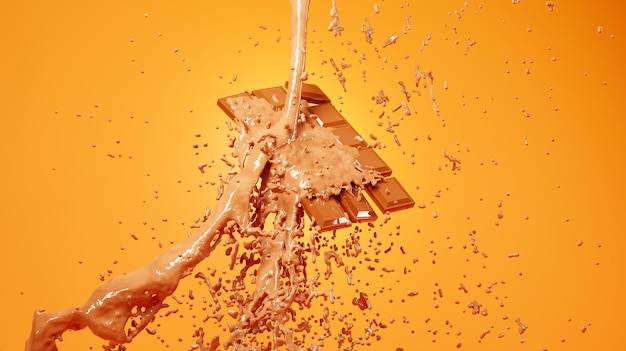This striking image features a dynamically staged scene with an orange background as its canvas. At the center, a chocolate bar composed of breakable square segments appears to hover in midair. The chocolate squares, particularly those at the top right corner and along the bottom edge, are visibly breaking apart. From above, a stream of chocolate milk cascades down, striking the bar and causing dramatic splatters and droplets to scatter in all directions. The liquid hits the chocolate bar around the middle, with some of the chocolate milk arcing off toward the bottom left, creating an action-packed visual effect. Light and dark shades of brown from the chocolate and milk, contrasted against the orange background, accentuate the intense, real-time moment captured in this photograph.